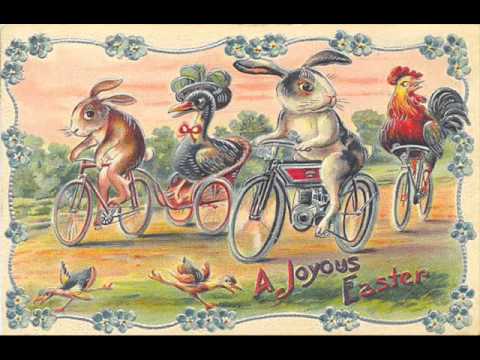The image is a charming, hand-sketched, colored pencil drawing reminiscent of a children's book illustration. It features four lively animals riding bicycles along a dirt path. On the left, a brown bunny pedals a bicycle, towing a small two-wheeled cart filled with a blue duck adorned with a red ribbon around its neck and a hat perched on its head. Following them, a gray bunny with a white stomach maneuvers a bicycle, while in the rear, a rooster with vibrant red, orange, and yellow feathers and a black tail rides his own bike. The scene unfolds under a pinkish-reddish sky, with trees and bushes sketched in the background. A wavy vine of greenish-blue with five-petaled bluish-green flowers frames the image, enhancing its playful, festive atmosphere. Along the path's yellow and brown hues, green grass borders the route, adding depth to the scene. Beneath this joyful parade, the words "A Joyous Easter" appear, surrounded by tiny birds and floral motifs, encapsulating the festive spirit of the illustration. The entire image is neatly contained within a rectangular frame, accentuated by thin black borders on the top and bottom.